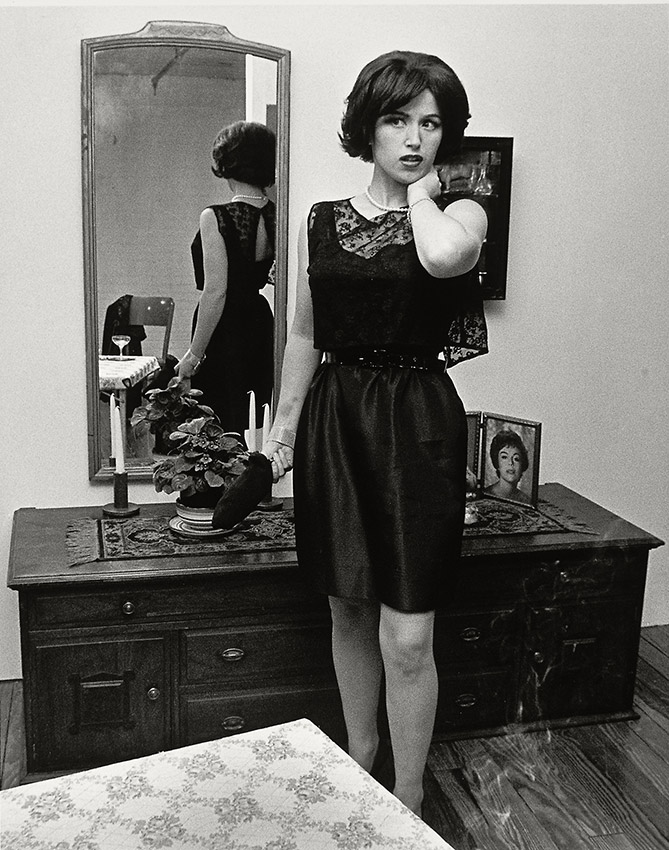This black-and-white photographic portrait captures a young white woman, likely in her late 20s to early 30s, standing indoors in front of a low, dark wooden dresser. She is attired in a short black dress paired with a black lacy blouse and accentuated with a white pearl necklace. Her short dark hair grazes just at her jawline. With her left hand gently placed on her neck, she holds an indistinguishable black object, possibly a clutch purse, in her right hand adorned with a prominent bracelet.

The dresser behind her features two sets of drawers and supports an assortment of items: two candles, a green potted plant, and a framed photograph of another woman. A wall-mounted mirror above the dresser reflects the back of her outfit, which has a slight opening, revealing her upper back. The mirror also catches a glimpse of a table set with a glass and a chair draped with a jacket. The floor beneath is hardwood, contributing to the classic ambiance of the scene. The intricate details and style suggest a bygone era, further underscored by the monochromatic tone of the photograph.